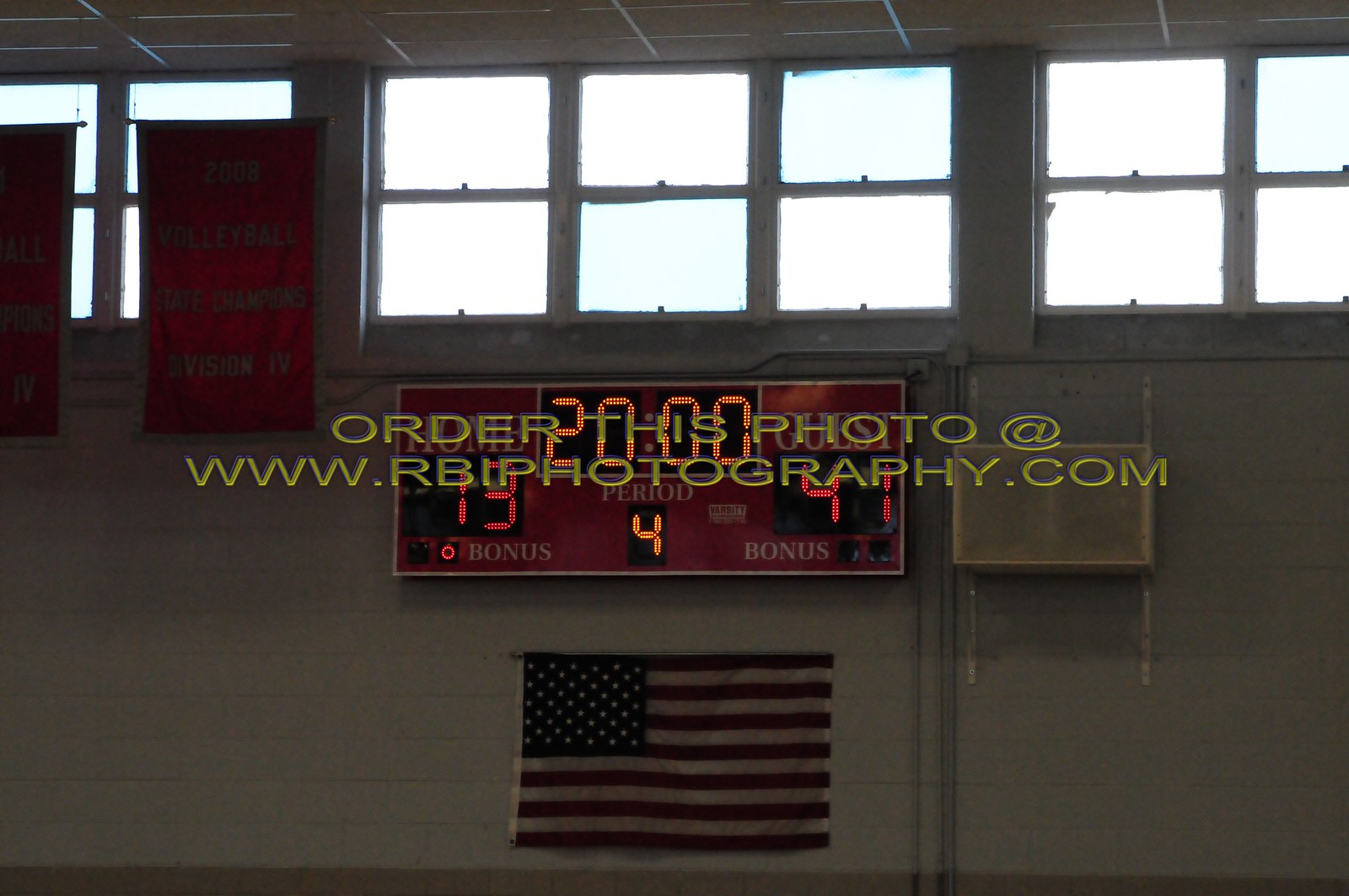The image is a photograph, likely captured with a disposable hand camera, evident from the general pixelation and film grain present. The lighting is very low, and an embossed gold watermark in the middle of the image reads, "order this photo at @ www.rbifotography.com." The photo is of a gymnasium scoreboard, prominently displaying scores and times. The home team score on the left is 13, lit up in red, while the guest team score on the right is 41, also in red. The middle clock shows 20 minutes, and the period number in gold is 4. Below the scoreboard hangs an American flag against a white brick wall. The top half of the image features large, foggy windows that allow light to pour in, with two red flags hanging from the ceiling in front of the windows on the left, though their details are obscured by darkness. The background of the scoreboard is red, accented with gold, and additional details, such as banners for previous accolades, are visible but not clearly readable due to the low light and watermark in the center.